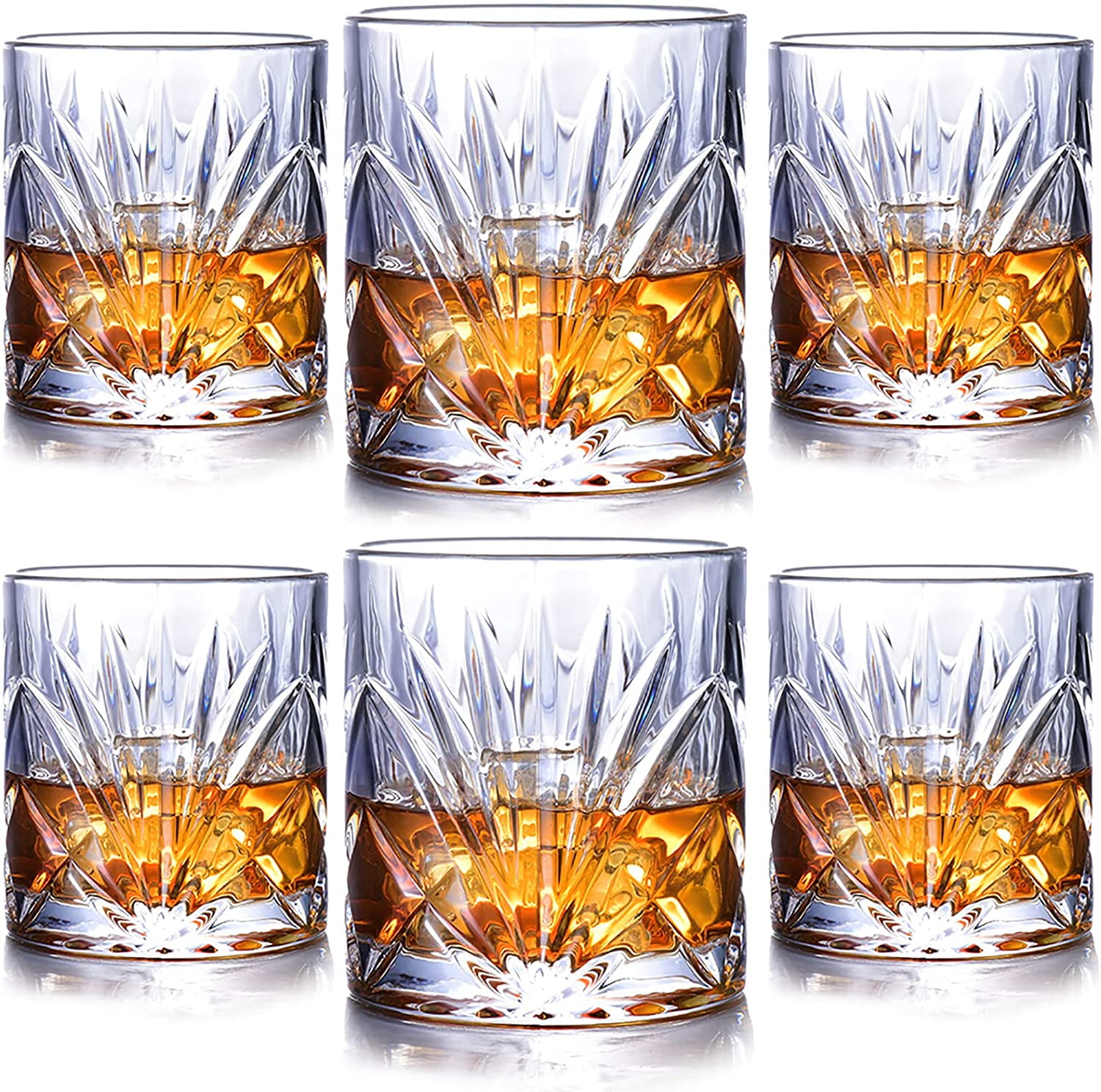The image showcases a close-up of six elegantly designed, clear crystal whiskey shot glasses, arranged with three glasses in the top row and three in the bottom row. Each row features a larger middle glass flanked by two smaller ones on both sides. All six glasses are uniformly half-filled with a rich, amber-colored liquid, presumably whiskey. The glasses have a distinctive, ornate cactus-like design etched into them, characterized by an angular, spiky pattern that adds a touch of sophistication. The backdrop is a subtle, pale white, enhancing the reflective quality of the glasses' surfaces and their intricate details. This careful arrangement and the elegance of the glasses suggest a refined setting, ideal for a distinguished party or gathering.